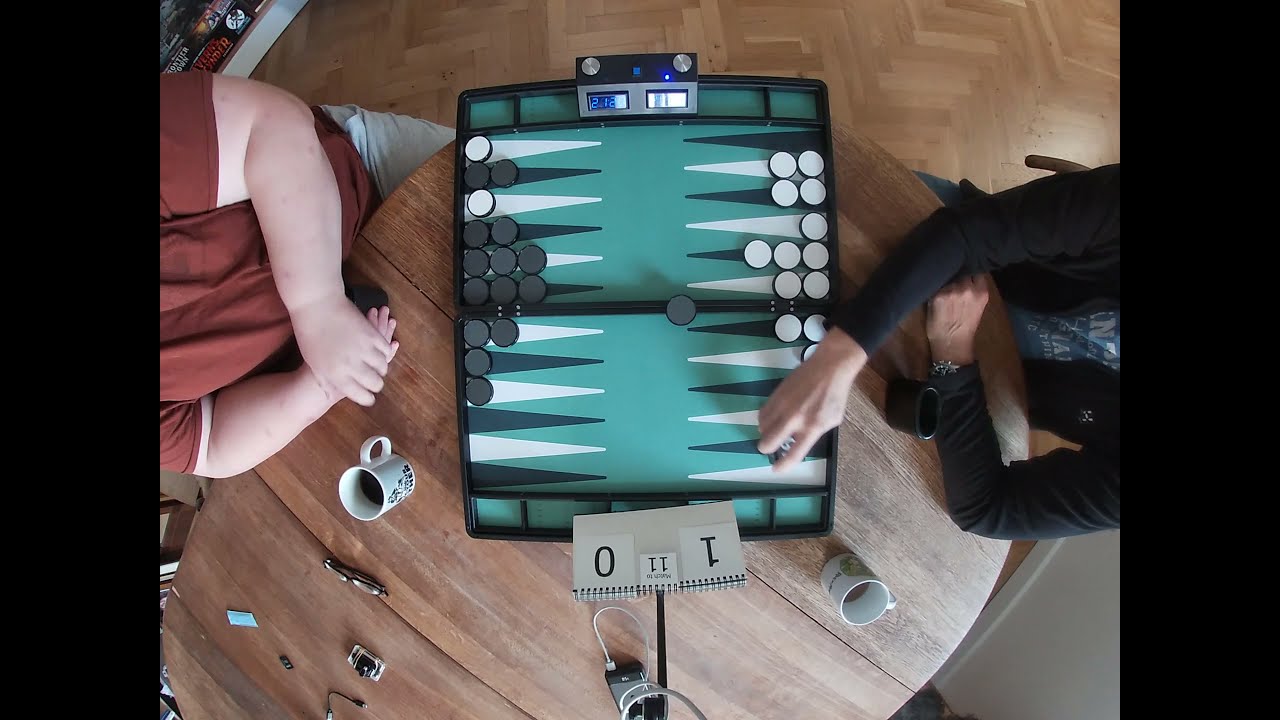An overhead photograph captures an indoor gaming scene where two people are engrossed in a game of backgammon on a round wooden table set on a wooden floor. The backgammon board, embellished with green, black, and white hues and adorned with round black and white checkers, is centrally placed. The player's faces are not visible; only their torsos and arms are in view. On the left, a slightly heavy-set individual wearing a short-sleeved burnt orange shirt and grayish pants has their hands folded. Their opponent on the right, possibly thinner, sports a dark gray long-sleeve shirt under a black jacket, accessorized with a watch. Each player has a coffee cup filled with liquid beside them. A manual scoreboard, featuring a sequence of numbers—1, 11, and 0—extends from a small hole at the bottom center of the table. The predominant colors in the image are green, black, white, tan, brown, red, gray, and silver. Black bars frame the left and right edges of the horizontal rectangular image, emphasizing the main action at the center.